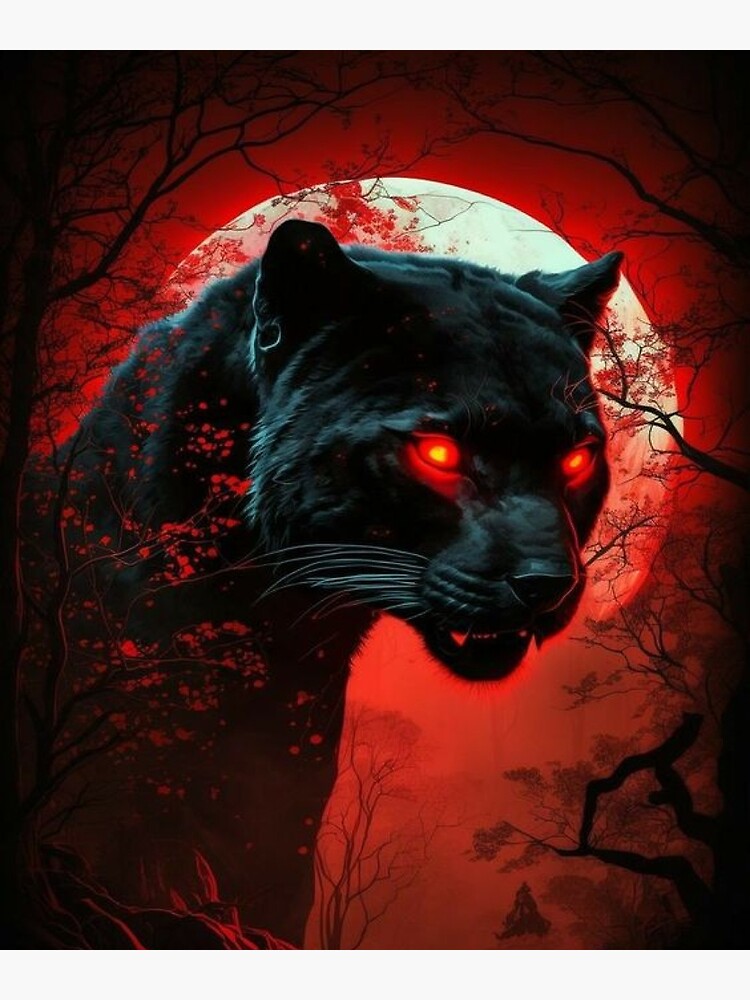The image is a pixel art piece depicted in predominantly shades of black, white, and red. It features a fierce black wildcat, resembling a panther, with its head and upper shoulders at the center. The panther's menacing eyes, glowing a fiery red with dark yellow centers, stand out against its dark fur. Red speckles, possibly indicating blood, pattern its neck and chest, adding to its ferocious appearance. Its white whiskers and sharp, partially revealed white teeth further accentuate its predatory aura. The background showcases a blood-red night sky with silhouetted black tree branches reaching inward from the edges towards a large, glowing white full moon that forms a halo around the panther's head. The image is vertically rectangular with very dark corners and faint borders at the top and bottom, emphasizing the central, dramatic scene.